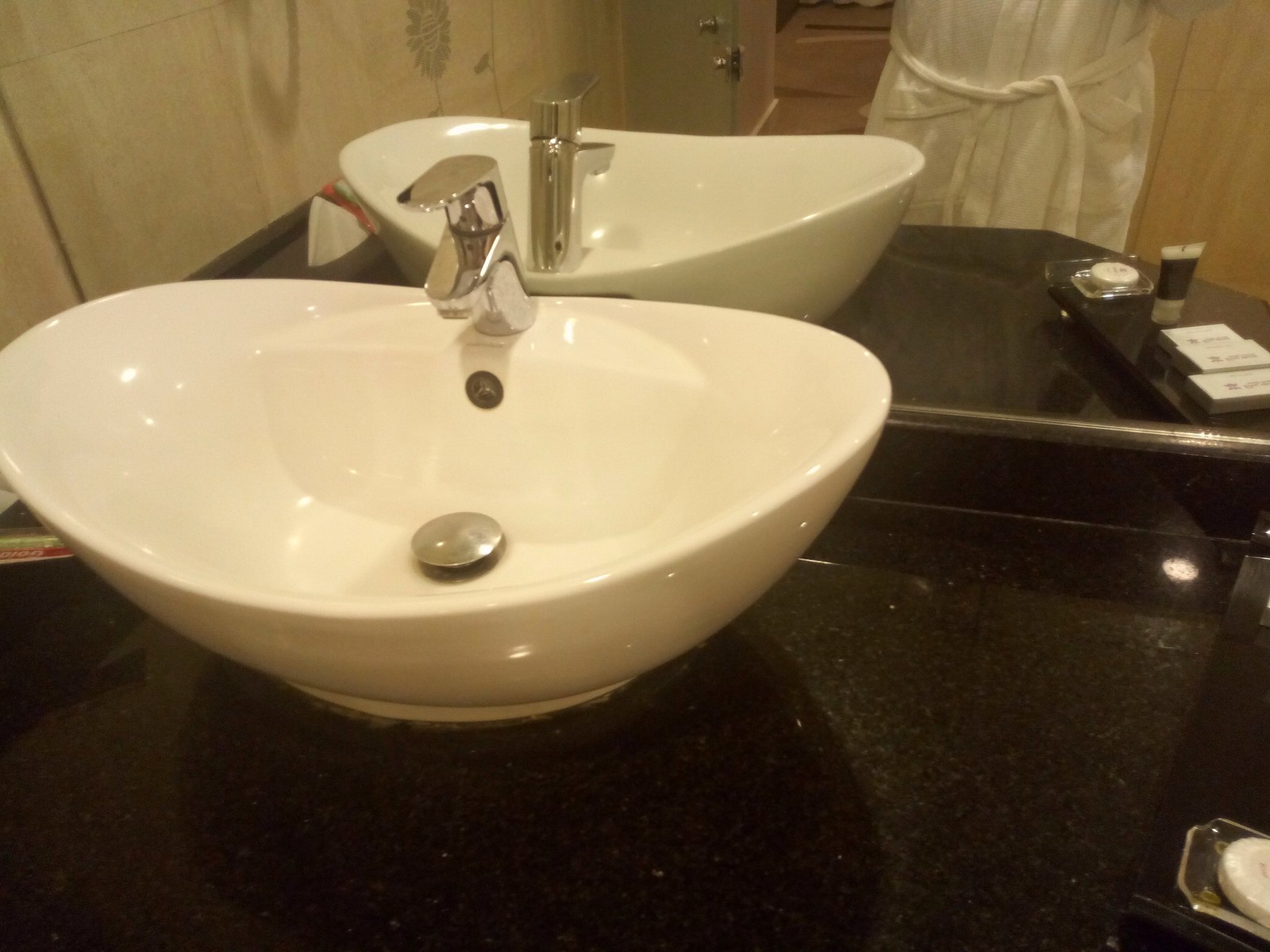This sepia-toned photograph captures a bathroom scene centered around an elegant, white porcelain sink with an above-counter, bowl-shaped design. The sink features a sleek, single chrome fixture with a lever handle, a steel stopper, and an overflow hole. Positioned on a striking black countertop, the surface appears slightly textured, adding a tactile element to the composition. In the mirror behind the sink, a person wearing a belted white robe is partially visible from the waist down, likely the photographer based on the angle. The countertop is not entirely barren; among the items present, there is a small container of lotion, a circular disc-shaped object on a glass pedestal, a bottle with a black band, white top and bottom, and three white boxes with indistinguishable text. An additional red item featuring the word "Colgate" can be seen in the upper left corner, though it is partially obscured. The overall arrangement creates a blend of reflective elements and functional items, highlighting both the practicality and aesthetic appeal of the space.